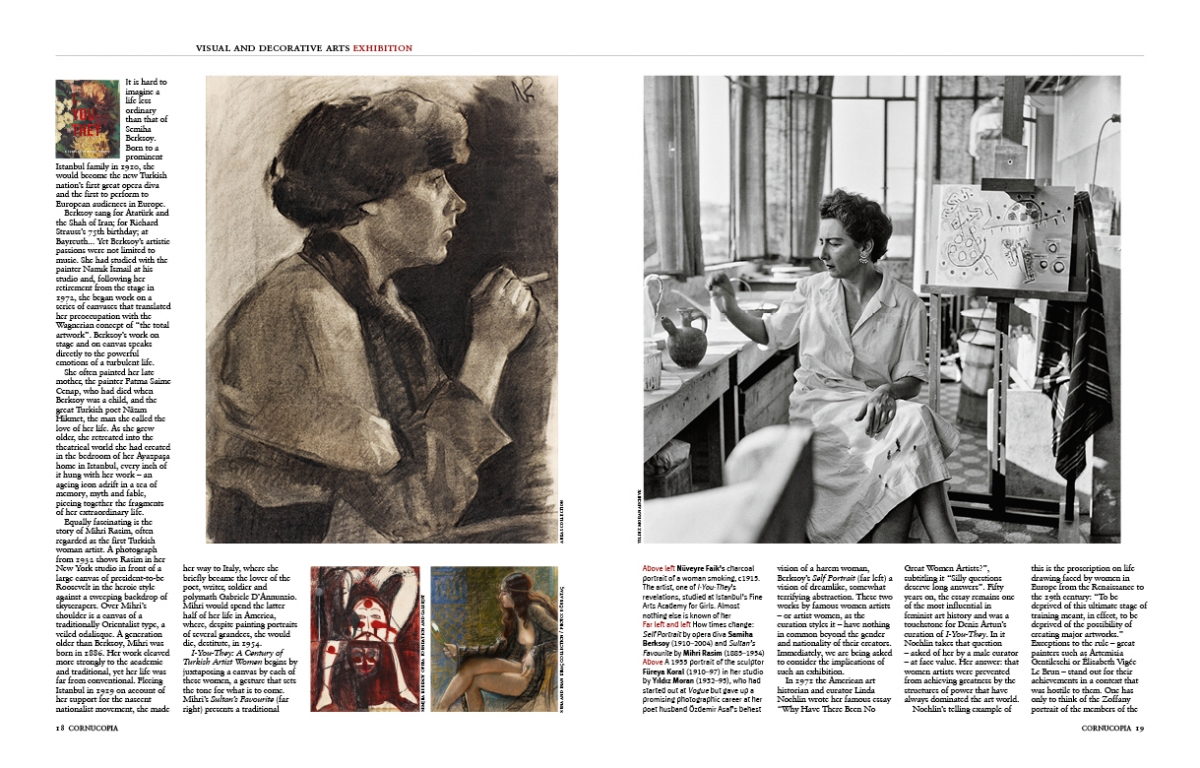The image displays a two-page spread from a magazine that features text and photographs presented on a white background. The left page consists of two columns of very small black text at the top, followed by a prominent, grayscale illustration of a short-haired woman wearing a scarf around her neck, holding a cigarette, and staring thoughtfully out of a window with her elbow resting on a table. Below this illustration, there is another column of text and two smaller pictures: one shows a small rectangular image of a flower or a floral vase, and another at the bottom right corner depicts a woman sitting in a chair. Across the two pages, various images and photographs are strategically placed to complement the text. The right page is dominated by a large black and white photograph in the center, featuring a woman in a white frock, engrossed in her pottery work inside a studio. Behind her are windows and a whiteboard with sketches on it. Beneath this central photograph are four columns of text. The spread appears to be from a magazine that focuses on visual and decorative arts exhibitions, as indicated by the faded header text at the top.